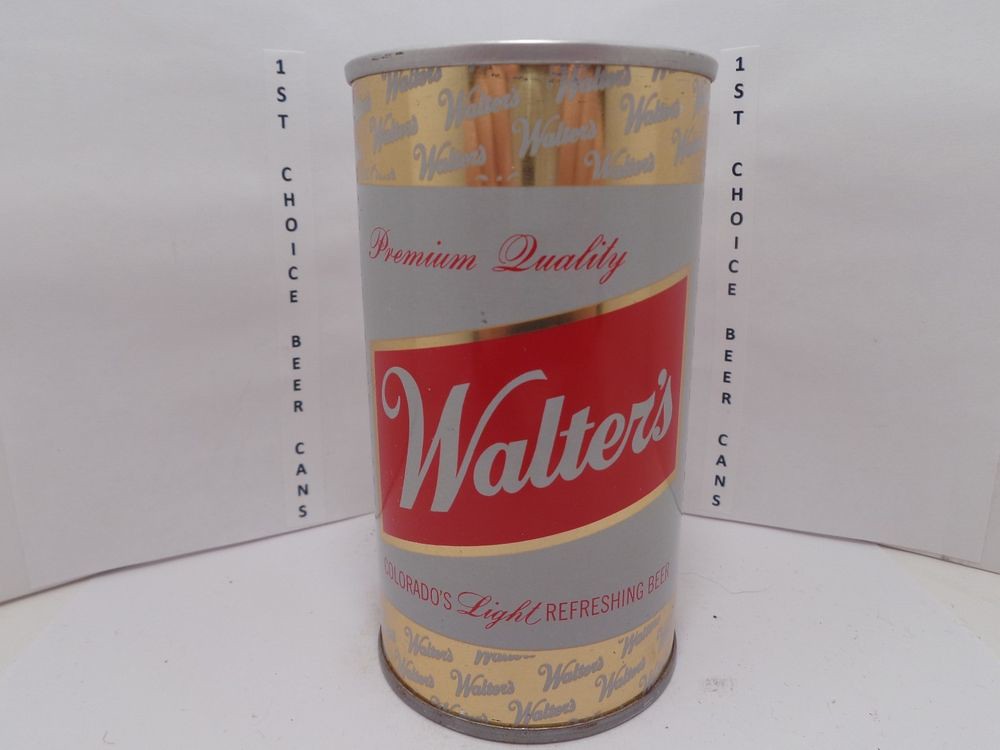This is an up-close photograph of a vintage beer can sitting on a white surface with a white background. The can features a distinctive design with multiple sections. At the top, there is a silver-colored rim followed by a reflective gold band with the word "Walters" repeated in gray. Beneath this, a white section bears the red cursive script "Premium Cup Quality." Below that, a thick red band is bordered in gold and contains "Walters" in white cursive letters. Further down, another white band features the red text "Colorado's Light Refreshing Beer." The can has a gold band at the bottom with "Walters" once more in gray script, and the very base of the can appears to be made of corroded and rusty stainless steel. The background wall prominently displays the vertical black text "1ST Choice Beer Cans" on both the left and right sides of the can. The can appears to be taller and narrower than contemporary beer cans, contributing to its vintage and possibly aged appearance.